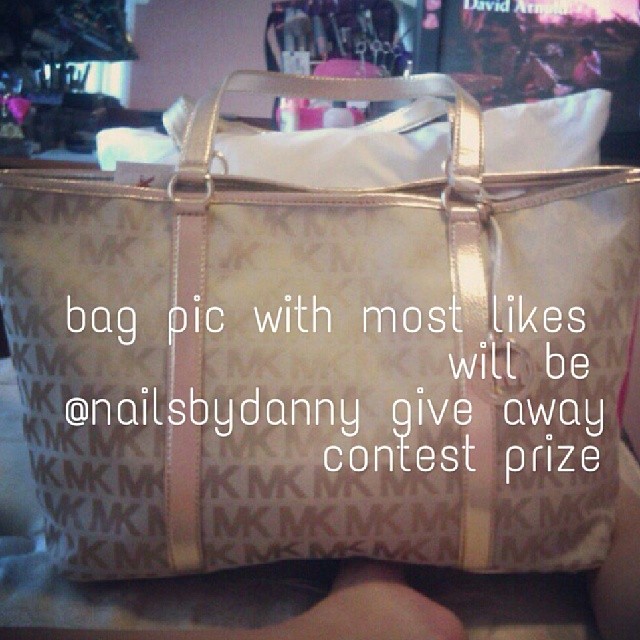This image is a detailed, color product photograph of a designer handbag, prominently gold in color, with the MK logo printed continuously across its fabric. The bag features shiny gold handles with brass round buckles connecting the handles to the body of the purse. The setting appears to be in a nail salon, subtly indicated by a visible booth in the background, designed for hand treatments. There is a touch of decor featuring pink roses in the top left corner. Over the image, white text reads, "Bag pick with most likes at Nails by Danny will be giveaway contest prize," styled mostly in lowercase and aligned to the right, adding a social media promotional aesthetic to the overall composition.